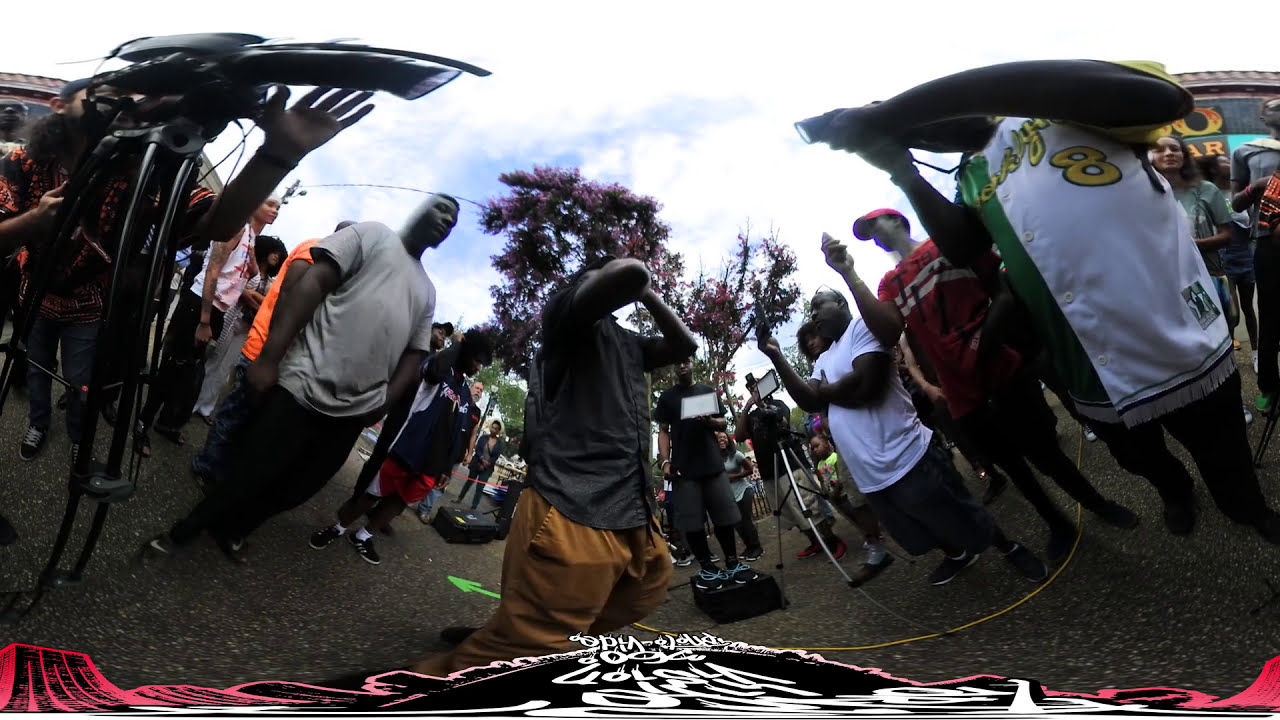The photo, taken with a GoPro or similar camera resulting in a curved and somewhat distorted view, depicts a large group of predominantly African or African-American individuals gathered outside on a road. The scene is set against a backdrop of a light blue sky dotted with large, puffy white clouds and the tops of trees, with hints of buildings on the periphery. The image is slightly blurry and gives an impression of being taken from the ground at eye level, adding to the distortion.

In the foreground, a man stands at the center of a crowd that forms a circle around him. He is wearing a dark charcoal gray, short-sleeved button-down shirt and brown khaki pants. With both hands clutching his face, he appears to be yelling something. The crowd is composed of individuals casually dressed in t-shirts, shorts, and pants, with a mix of men and a few women. Some members of the crowd are holding high-tech video cameras or cell phones, recording the central figure, while others are simply observing the scene. The image captures a dynamic and chaotic atmosphere, highlighting the collective focus on the man in the middle.